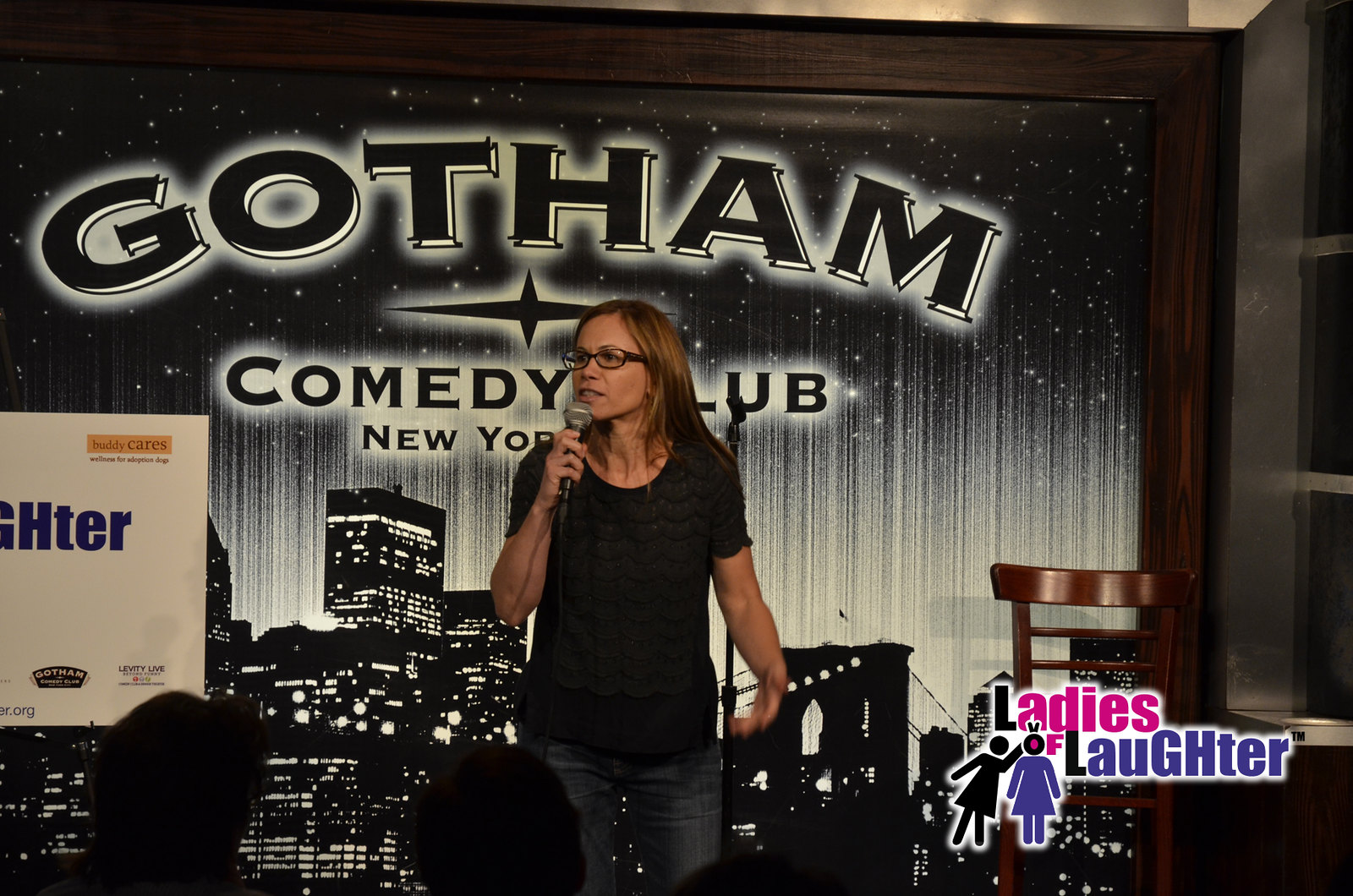This image features a middle-aged Caucasian woman with tan skin, wearing black-framed glasses and a black loose-fitting top paired with blue jeans. She has straight light brown hair falling just below her shoulders. The woman is captured mid-performance, holding a microphone with a black base and silver head, onstage at the Gotham Comedy Club in New York City. She is looking to her right, exuding a confident and engaging presence. Behind her, the club's iconic black-and-white sign displays the words "Gotham Comedy Club, New York" in a bold serif font, with a stylized depiction of the New York City skyline, including recognizable structures like the Brooklyn Bridge. The backdrop further features black-and-white streaks with scattered white dots, enhancing its dynamic visual appeal. Additionally, on the bottom right of the background, the logo "Ladies of Laughter" appears in pink and purple letters, accompanied by images of two stick-figure women, hinting at a comedy event focused on female performers. The silhouettes of several audience members' heads are visible at the bottom of the frame, suggesting a lively and attentive crowd.